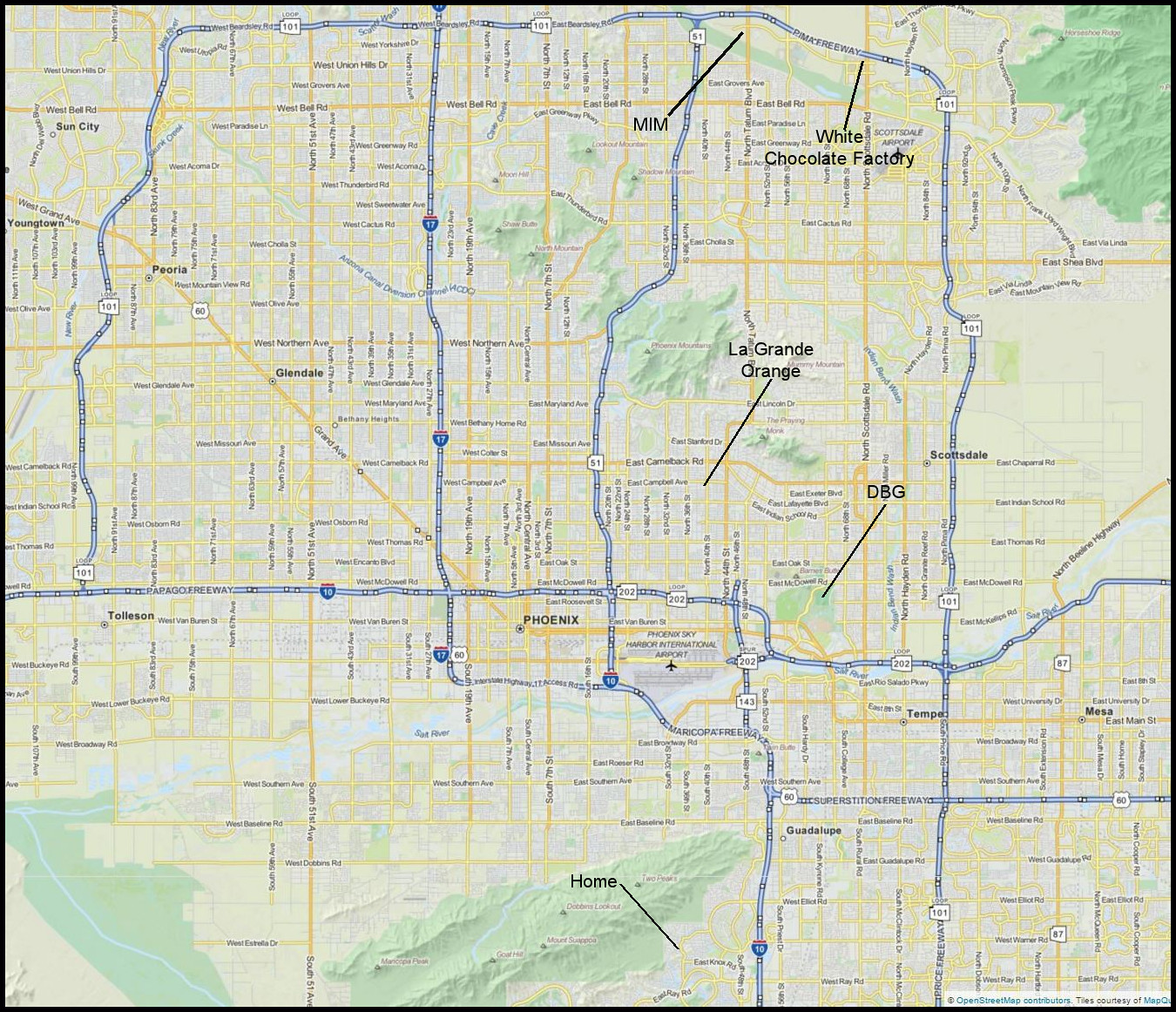The image depicts a detailed map on a white background featuring various colors indicating different elements. Prominent blue rectangular lines, some straight and others wavy, traverse the map. One specific blue line starts at the bottom right corner and extends upwards, then turns left towards the top left, and finally descends.

Yellow lines crisscross the map horizontally and vertically, likely representing streets, with lighter yellow lines inside them indicating residential districts. Several labels in black text annotate notable locations on the map. 

In the top right corner, "White Chocolate Factory" is labeled with a diagonal black line pointing to a blue line. Nearby, another diagonal line points to the acronym "MM". Central to the image, "La Grande Orange" is marked with a similar black diagonal line pointing towards the map's middle. Below and slightly to the right of La Grande Orange, "DBG" is located.

Smaller text annotations indicate locations in the surrounding areas: "Sun City" at the top left, "Peoria" in the middle left, "Glendale" on the bottom right, as well as "Mesa" and "Temple" in the bottom right. Centrally at the bottom, "Phoenix" is labeled in black text. This map provides a detailed view, highlighting key landmarks and geographical divisions.